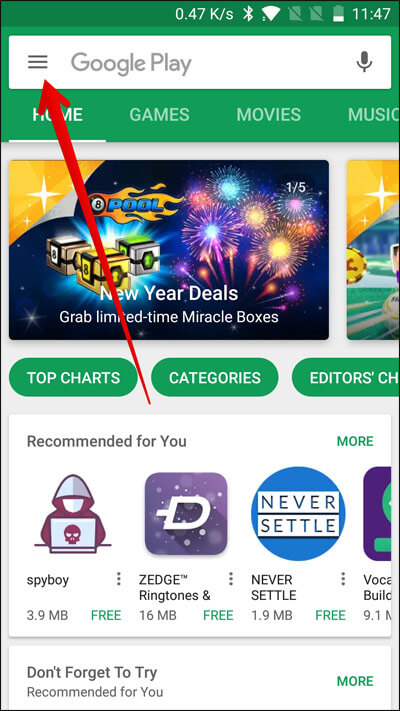Screenshot of Google Play Store Mobile Interface:

The screenshot captures the Google Play Store in a mobile view. The header at the top is green, showing vital information. At the very top, you see "0.47K/s" followed by various symbols, including a battery icon that appears about 25% full. The time displayed is 11:47.

Below the header is the search bar area, featuring three horizontal lines (hamburger menu) on the left, the text "Google Play," and a microphone icon on the right. Immediately under this, there's the navigation bar with categories listed: "Home," "Games," "Movies," and "Music." A thin white line is visible beneath "Home," but not directly under it.

Beneath the navigation bar, there is an advertisement presented in a rectangular banner. The ad promotes "New Year Deals" with the tagline "Grab Limited Time Miracle Boxes." The illustration includes fireworks and boxes labeled with numbers.

Following the advertisement, another navigation bar appears, this time with rounded buttons labeled "Top Charts," "Categories," and "Editor's Choice" (with the last word partially cut off). The section below this is titled "Recommended for You" and displays icons for various games such as "Spy Boy," "Zedge," "Ringtones," and "Never Subtle."

At the very bottom, there's a prompt saying "Don't Forget to Try," followed by another "Recommended for You" section with a green "More" button in the bottom-right corner.